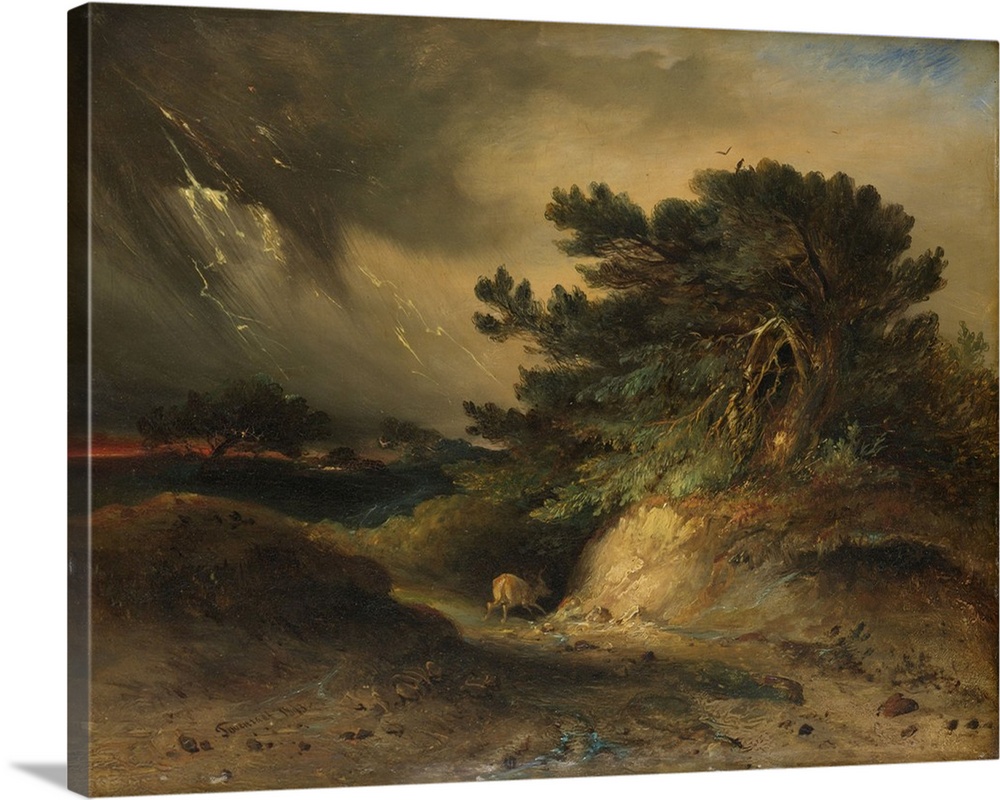The image showcases a painting on a canvas viewed from a three-dimensional angle. The canvas, tilted slightly to the right, reveals its left side, emphasizing its tangible texture and material. The painting itself depicts a tempestuous, stormy scene. The top left of the painting is dominated by violent grey clouds, rainfall, and striking bolts of lightning. Below, clusters of old trees appear chaotic, their leaves scattered wildly, suggesting the presence of strong winds. The trees’ branches are contorted and swaying, evidently affected by the storm. In the bottom center of the painting, a deer is shown in mid-run, seeking refuge in a crevice nestled in the hills of the forest. The deer’s urgency highlights the encroaching storm clouds from both the left and the right. Despite the looming tempest, patches of clear sky on the right hint at the impending engulfment by the swiftly advancing storm.